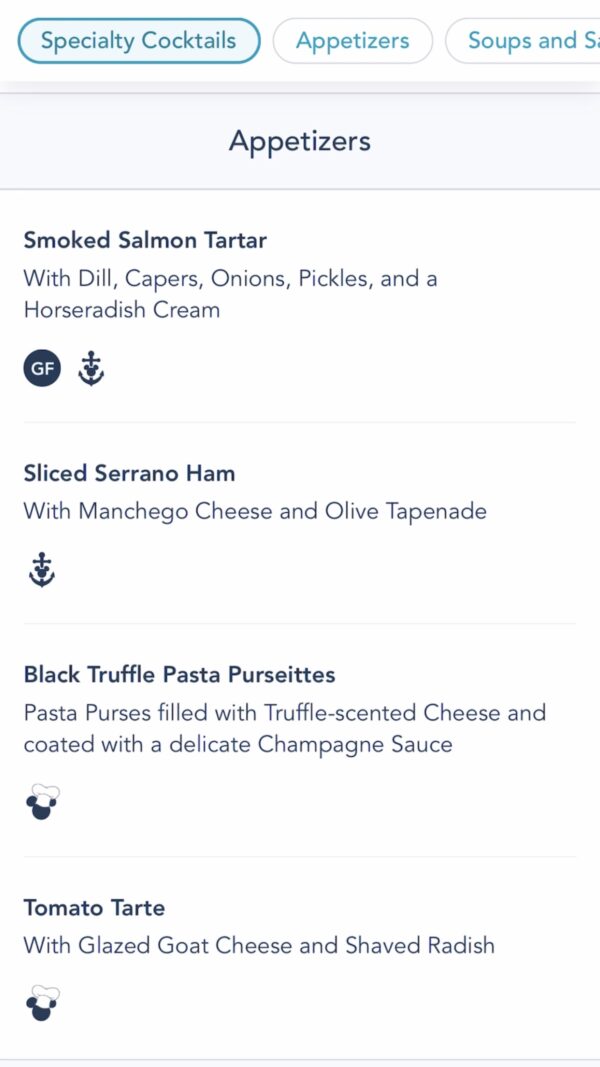This screenshot features the appetizers menu section from a dining establishment, likely aboard a Disney cruise, as evidenced by the presence of nautical Disney icons. The menu is neatly organized with tabs at the top for various categories such as Salty Cocktails, Appetizers, Soups, and Salads, with the Appetizers tab currently selected.

Under the Appetizers heading, four dishes are detailed with descriptions and icons indicating dietary information and chef recommendations. The first appetizer is Smoked Salmon Tartare, made with dill, capers, onions, pickles, and horseradish cream. It is marked as gluten-free (GF) and features an anchor symbol and Mickey ears, suggesting it is either a seafood dish or a chef's special.

The second item is Sliced Serrano Ham accompanied by Manchego cheese and olive tapenade, also adorned with an anchor symbol, potentially indicating a seafood dish or a chef's special.

The third appetizer listed is Black Truffle Pasta Persiettes, described as pasta purses filled with truffle-scented cheese and coated with a delicate champagne sauce. This dish is marked with a chef's hat featuring Mickey Mouse ears, denoting it as a chef's recommendation or special.

The final appetizer is a Tomato Tart topped with glazed goat cheese and shaved radish, also marked with a chef's hat and Mickey Mouse ears, indicating it is a chef's recommendation or special dish.

The overall design of the menu is clean and modern, with a white background and blue text. Icons provide clear information about each appetizer, catering to dietary preferences and highlighting special items with ease.